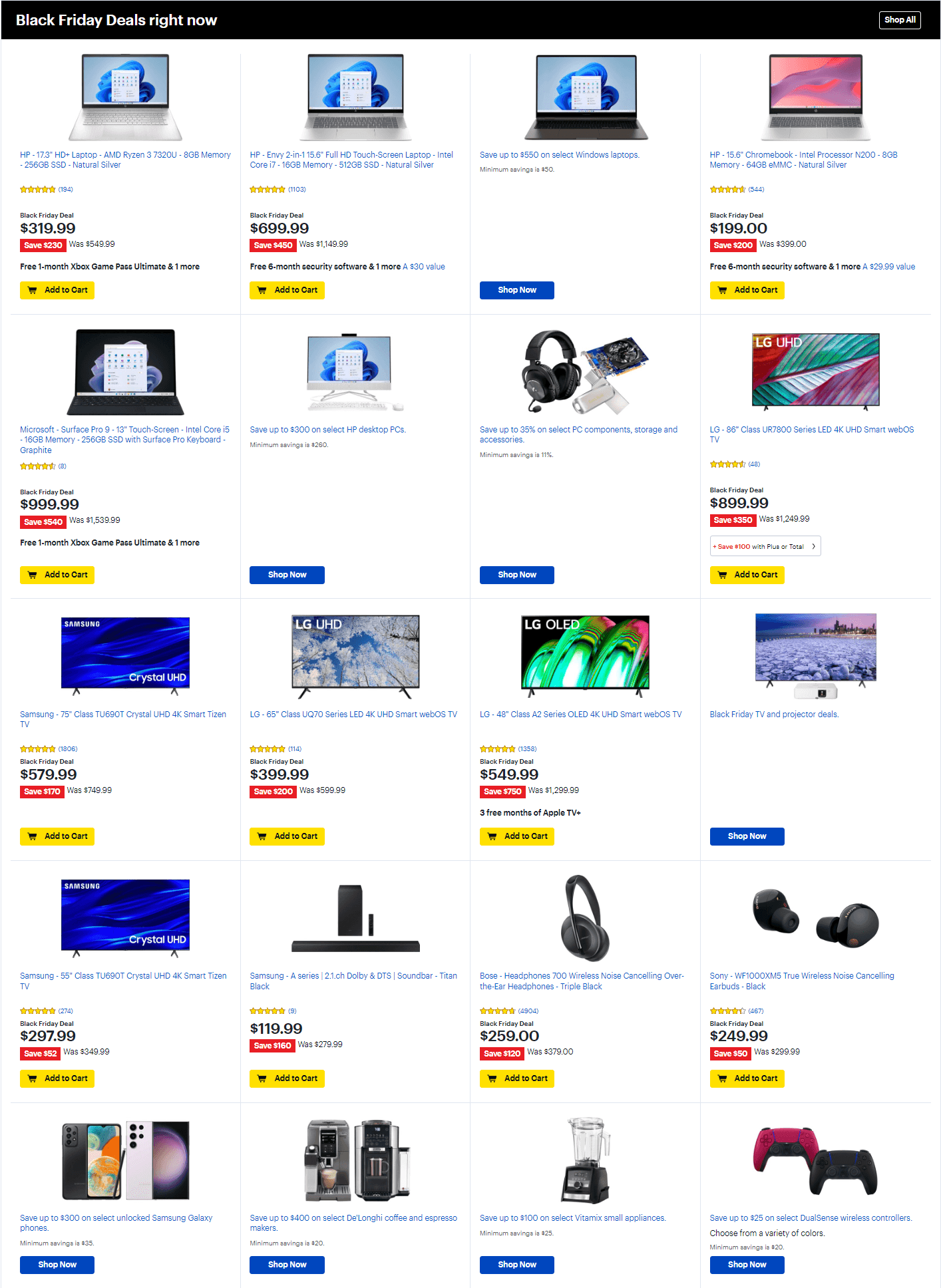This image is a comprehensive screenshot showcasing numerous Black Friday deals. It is notably long and contains detailed promotional content. At the top of the screenshot, a black banner spans from the upper left corner to the upper right corner, with the text “Black Friday Deals Right Now” on the left and “Shop All” on the right.

The screenshot is organized in a grid format with five rows and four columns of product images. Each image represents a different deal available for Black Friday. 

1. The image in the upper left corner features an HP laptop. However, this part of the screenshot is blurry, making specific details difficult to read. The laptop is priced at $319.99, accompanied by a red rectangle indicating the savings, and an orange "Add to Cart" button.
   
2. Next to it, in the first row, the second image also has an "Add to Cart" button, but no detailed description is provided.
   
3. In the first row, the third image has a "Shop Now" button, without additional information.

4. The image in the upper right corner of the first row displays another HP product priced at $199, showing savings of $200, and also includes an "Add to Cart" button.

All product images are part of the Black Friday promotions and highlight the savings in red text. Most images feature yellow "Add to Cart" buttons, suggesting a quick purchase option to capitalize on the limited-time deals. The emphasis on the ease and urgency of purchasing implies these deals might sell out rapidly.

The overall intent of the screenshot appears to be to entice shoppers with significant discounts and facilitate quick purchases during the Black Friday event.